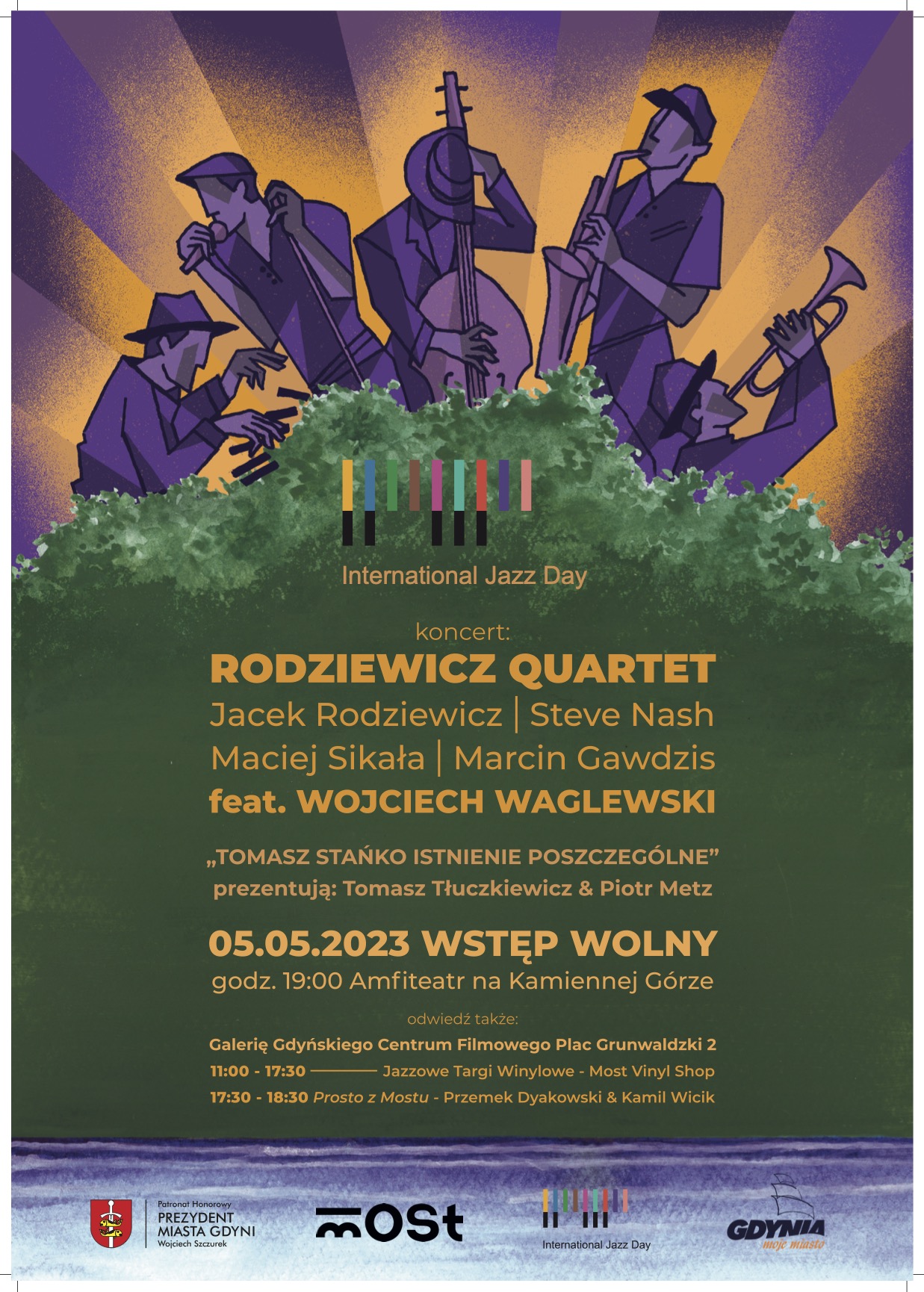This is an image of a poster for International Jazz Day Concert featuring the Ruzhik Quartet. The poster depicts five minimalist-styled, purple cartoon musicians with yellow rays radiating behind them on a purple background. Each musician is playing a different instrument: one on a piano, one with a microphone, one with a violin, one with a saxophone, and one with a trombone. The main text is placed in front of a large green bush, highlighting the yellow details of the event: "International Jazz Day Concert, Ruzhik Quartet featuring Jazzyk Ruzhik, Steve Nash, Ajik Siktada, Marcin Gajus, and Wojcik Pogorzelski." The concert is scheduled for May 5th, 2023, at 19:00 at the Amphitheater of Comfort. The poster also lists several sponsoring companies at the bottom and features additional show times. The Polish town of Wstęp Wolny is noted on the poster, indicating the location of the event.